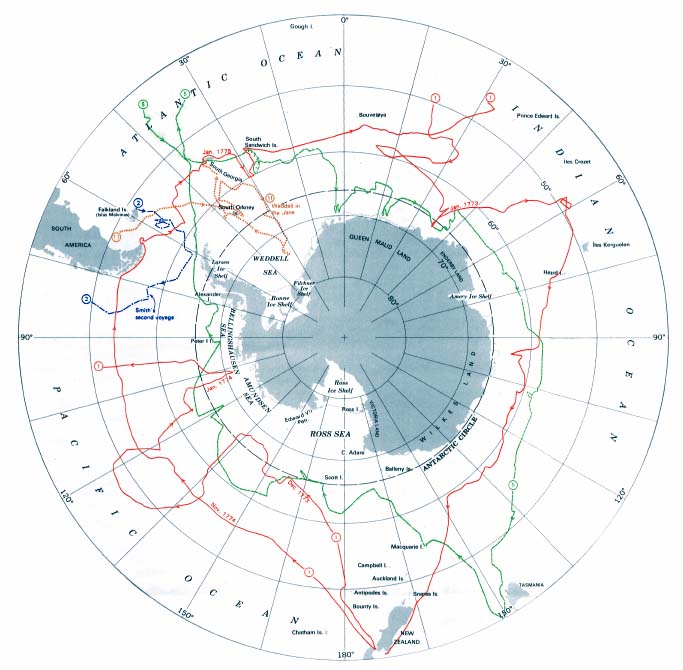This is a detailed circular illustration focusing on the Antarctic region with the South Pole at its center, giving a unique perspective of the world. The map highlights Antarctica prominently at the center, surrounded by the Atlantic, Indian, and Pacific Oceans. Radiating from the South Pole are lines with degree markers that help plot courses and possible routes. Notable in the top left quadrant is the visible tip of South America, adding geographic context. The map features various colored lines—green, red, orange, and blue—likely representing different voyages or routes. While primarily gray and white, the map includes labels identifying significant oceans and nearby regions, juxtaposing the bluish-gray hue of Antarctica with the stark white of the surrounding seas. The detailed depiction of the map lines, coupled with the central placement of Antarctica, truly turns conventional worldviews upside down.